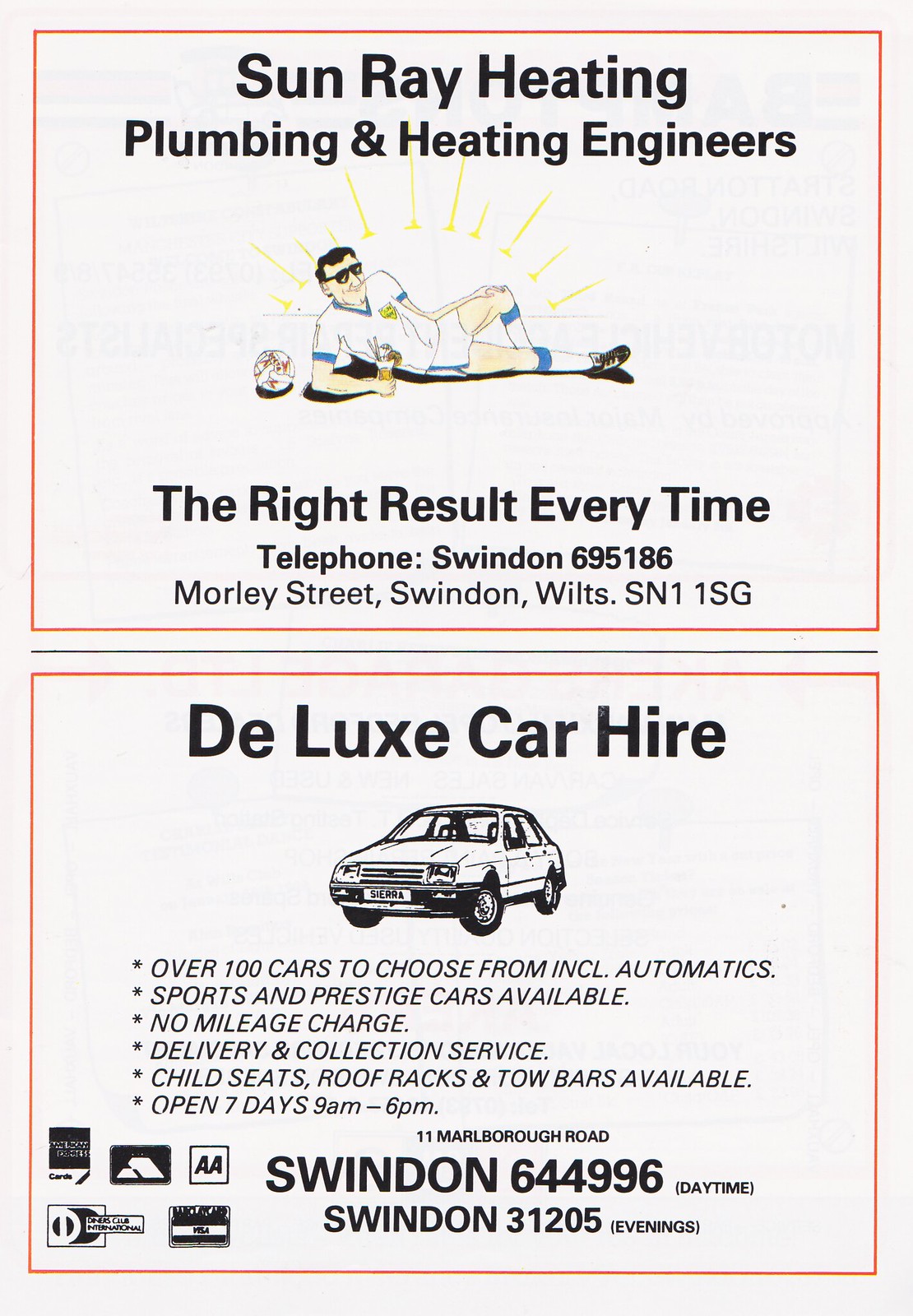The advertisement flyer is divided into two sections, with the top half promoting Sunray Heating, Plumbing, and Heating Engineers, and the bottom half advertising Deluxe Car Hire. The top portion features a white background with black text and includes a detailed illustration of a man lounging comfortably on a soccer field, dressed in a full soccer outfit complete with sunglasses and soccer cleats. He is casually holding a margarita-like beverage with a straw and an umbrella, with the rays of the sun casting a warm glow behind him. The text provides the company's slogan, "The right result every time," and details its contact information: Telephone Swindon 695186, located at Morley Street, Swindon, Wilts, SN1 1SG.

The lower section of the flyer advertises Deluxe Car Hire, highlighting a wide array of benefits such as having over 100 cars to choose from, including automatics, sports, and prestige models. It offers additional services like no mileage charges, delivery and collection, child seats, roof racks, tow bars, and operates seven days a week from 9 a.m. to 6 p.m. The contact numbers are Swindon 644996 for daytime inquiries and Swindon 31205 for evenings. An illustration of an old-style car is present, and the flyer displays various accepted payment methods, including American Express and Visa, in the bottom left corner.